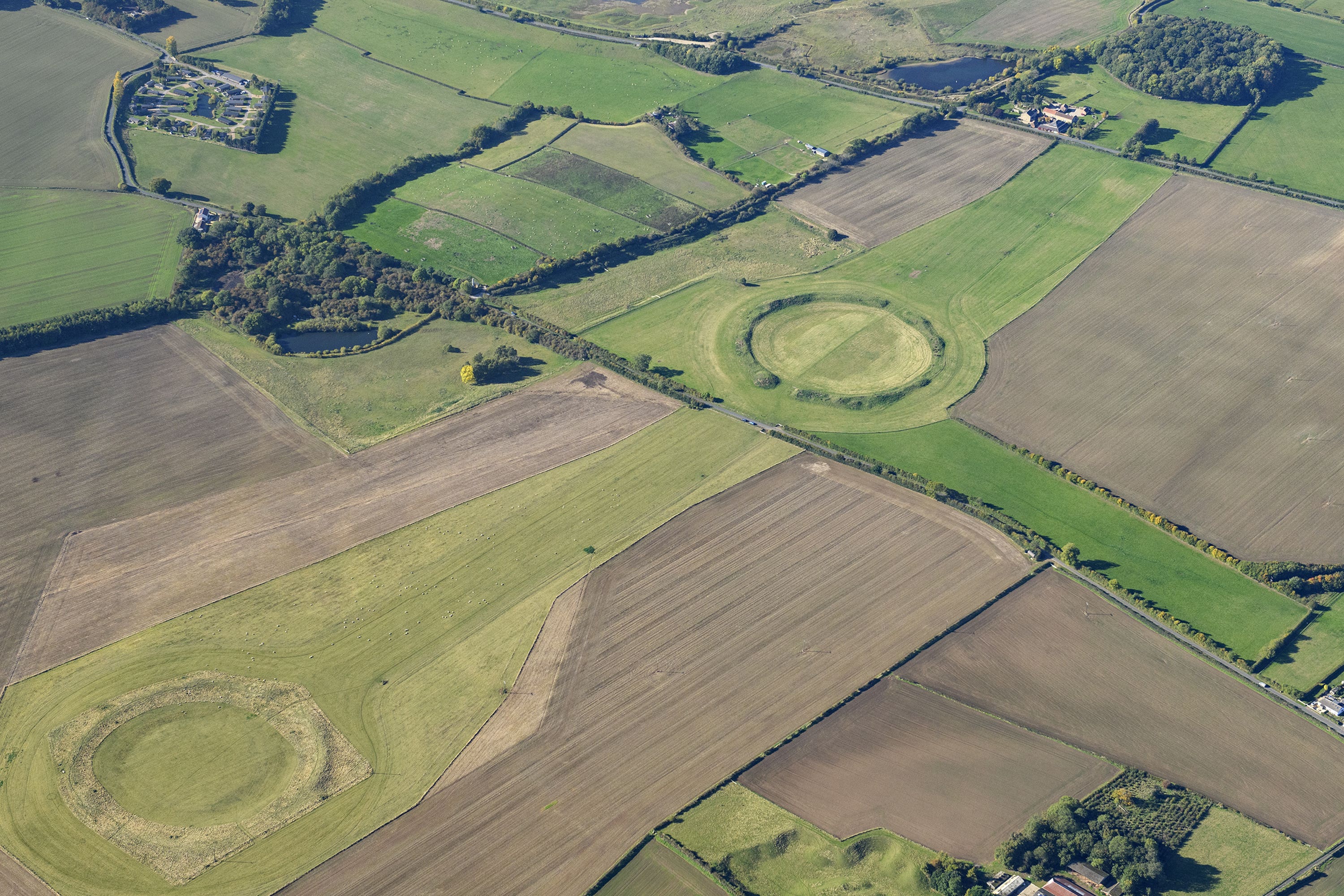This aerial photograph, likely captured by a drone, offers a sweeping view of expansive fields segmented into rectangular patches, separated by thin rows of vegetation or possibly brush. The landscape showcases a variety of textures and colors, with substantial areas of plowed brown fields, interspersed with wide stretches of green fields in various growth stages. Particularly notable are the intriguing circular formations scattered throughout the image, which appear meticulously maintained and distinctly green, possibly raised or outlined with vegetation. In the upper left corner, a denser clump of trees forms a circular area surrounded by lighter green terrain, further leading into smaller circular features and transitioning into more brown fields. The fields radiate neat, symmetrical lines, with orderly sections of trees contributing to the well-manicured appearance. Additionally, a small cluster of houses is visible in the top left, hinting at a diminutive neighborhood amidst this predominantly agricultural vista.